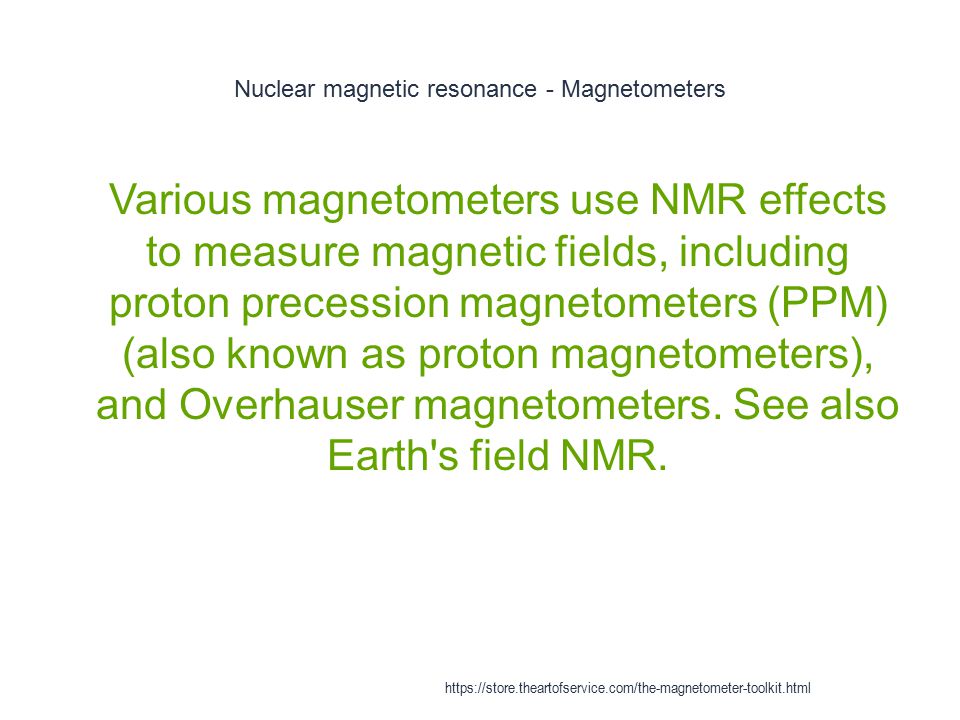The image appears to be a slide from a lecture or presentation with a white background. At the top, in small black text, it reads "Nuclear Magnetic Resonance - Magnetometers." Below this, centered on the slide, is a detailed explanation in medium-tone lime green text: "Various magnetometers use NMR effects to measure magnetic fields, including Proton Precession Magnetometers (PPM), also known as Proton Magnetometers, and Overhauser Magnetometers. See also Earth's field NMR." At the bottom of the slide, in small navy blue text, is a hyperlink: "https://store.theartofservice.com/the-magnetometer-toolkit.html."